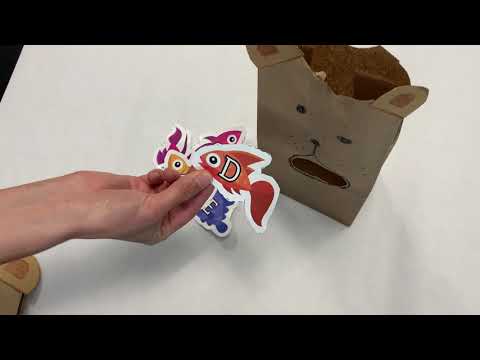The image is a close-up, color photograph in landscape orientation, capturing a person’s hand prominently in the center. The hand holds several vividly colored paper cut-out fish stickers, each outlined in white. The most noticeable fish is orange and marked with a capital letter "D" in a white uppercase serif font. Other visible fish stickers include a yellow one resembling a fish's nose, a pink fish, and an indistinct blue sticker partially hidden behind the orange fish. These stickers appear to be intended for a crafting project. Below the hand, set on a white tabletop, stands a reconfigured brown paper bag that has been artistically transformed to resemble an animal, likely a panda bear. The paper bag features ears crafted from its top corners and a face drawn in black marker, complete with expressive eyes, a nose, and a mouth. A beige element is partially visible on the table, obscured by the person’s hand. The scene suggests an engaging and creative activity in progress with a stylized and realistic photographic presentation.